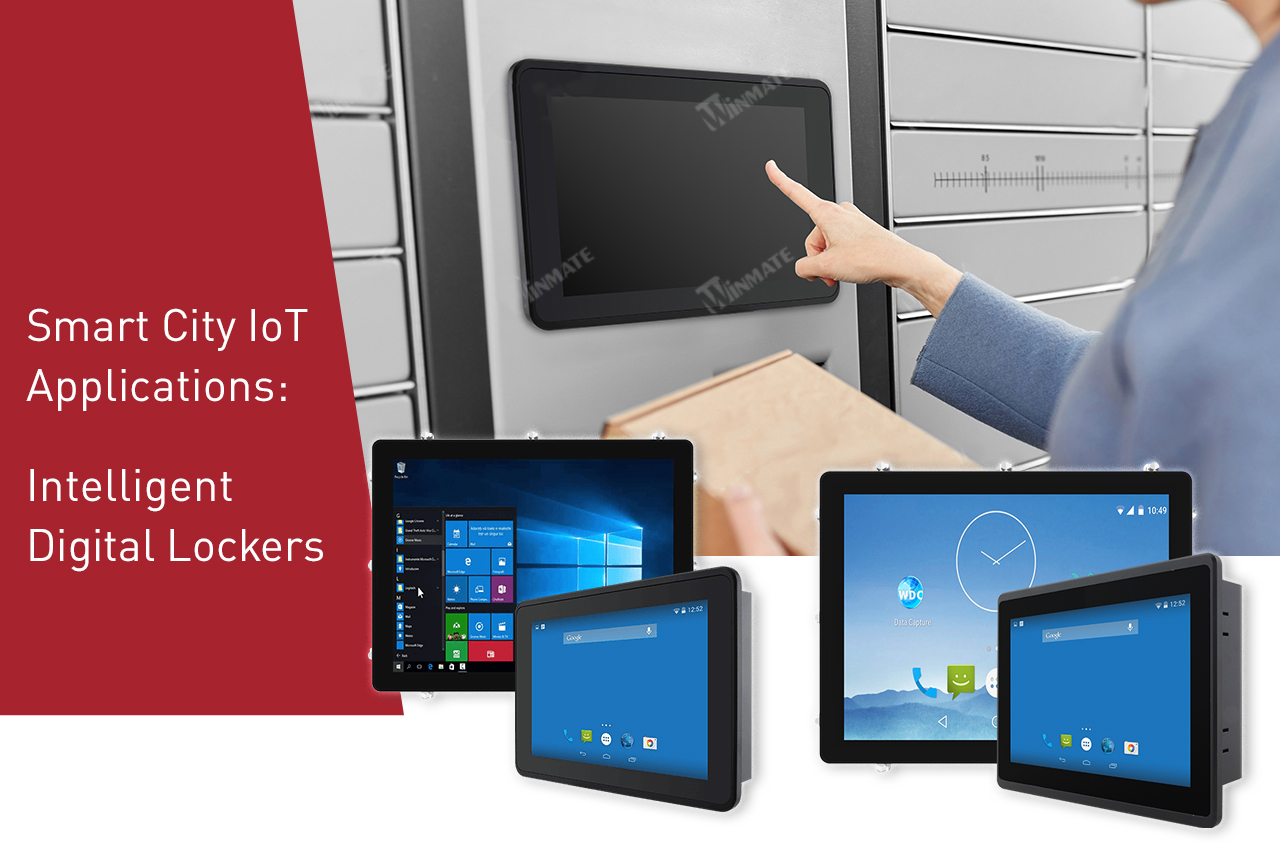The image is a horizontal rectangular advertisement showcasing Smart City IoT Applications and Intelligent Digital Lockers. At the center of the composition, a black tablet screen is mounted on a gray wall. A person, with light skin, dressed in a gray long-sleeved suit jacket, is seen extending their arm, with their finger touching the tablet screen, appearing to interact with it. On the left side of the image, a dark red stripe features white text that reads "Smart City IoT Applications, Intelligent Digital Lockers."

Beneath this text, there are several black-mounted display screens of varying sizes, each displaying blue interfaces. There are five screens in total, with four active ones positioned at the bottom of the image. The colors that dominate the image include gray, black, blue, red, and white. The exact placement and interaction of the elements create a clean and modern feel, although it's difficult to determine if the scene is a real photograph or a digitally created rendering to promote the digital lockers.